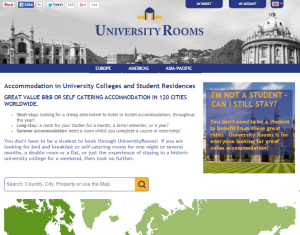"An advertisement for 'University Rooms' is prominently displayed at the top of the image. The headline reads 'Accommodations in University Colleges and Student Residencies', with a subheading promising 'Great Value or Self-Catering Accommodations in 120 Cities Worldwide'. The background of the advertisement features architectural landmarks that bear a resemblance to the White House or other significant monuments. Below the main text, in smaller white print on the right side, it reads: 'I'm not a student, can I still stay? You don't need to be a student to benefit from these great rates. University Rooms is for everyone looking for great value accommodations.' Further down, there is a map along with a search bar where users can input queries by country, city, or property. The search bar is accompanied by a yellow button with a navy magnifying glass icon. At the top section of the interface, there is a clickable area labeled 'Americans' among other options."